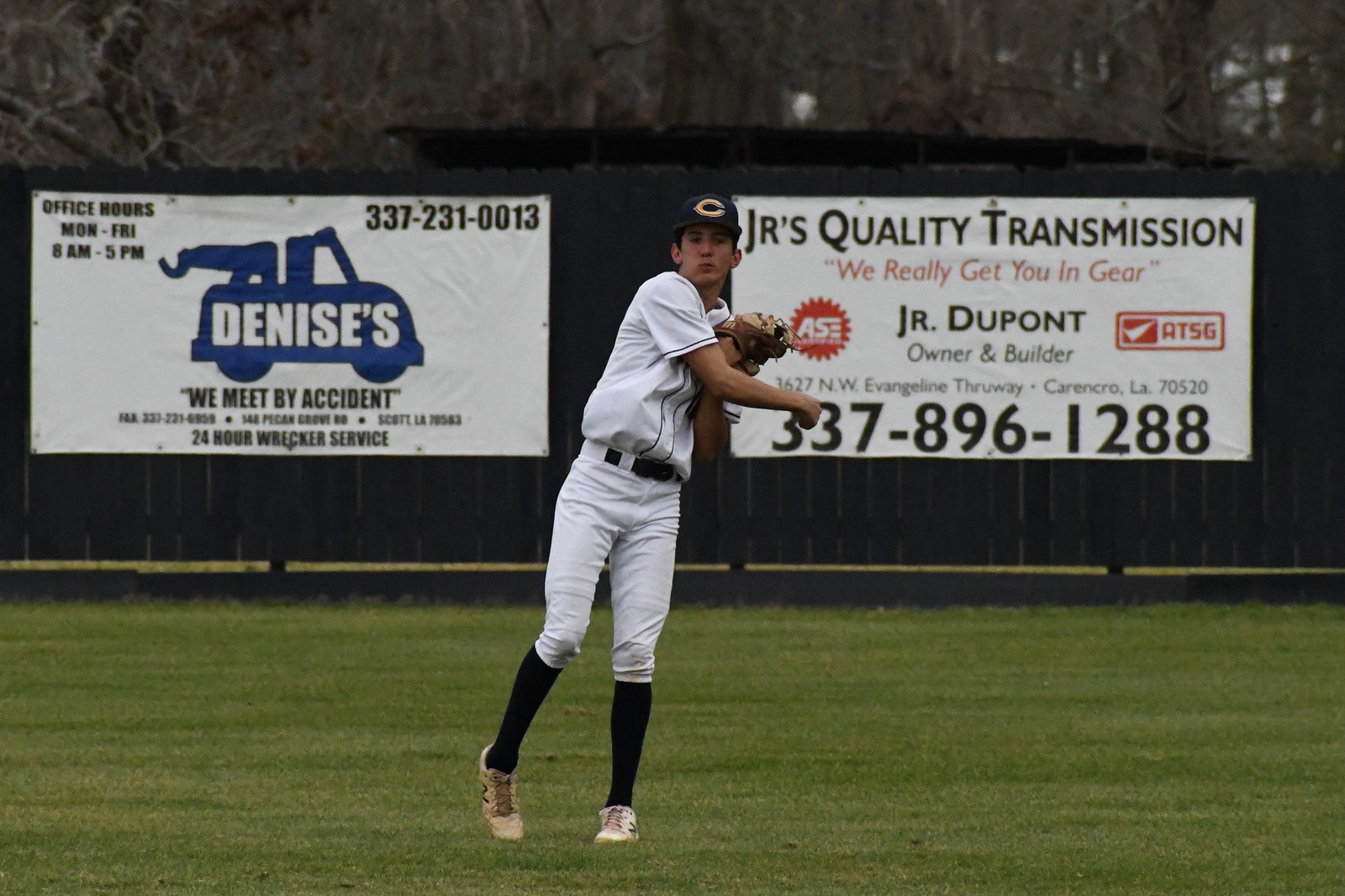In this detailed image, we observe a baseball scene set in a green grassy field under the bright daylight. At the center stands a young male baseball player who seems to have just thrown a ball, captured mid-motion. He is attired in a white jersey, white pants, black socks, beige cleats, and a black cap adorned with an orange "C" emblem, reminiscent of the Cincinnati team logo. 

Directly behind the player, an outfield wall prominently displays two large advertisements. On the left, a poster for Denise's depicts a blue tow truck and reads, "We meet by accident," indicating a 24-hour wreck service, with additional details including office hours and a contact phone number, 337-231-0013. On the right, an advertisement for Junior's Quality Transmission boldly states, "We really get you in gear," listing Junior DuPont as the owner and providing the phone number, 337-896-1288.

The rich array of colors in the image—green, black, white, blue, red, brown, and yellow—accentuates the vibrant and dynamic setting of this baseball field scene.